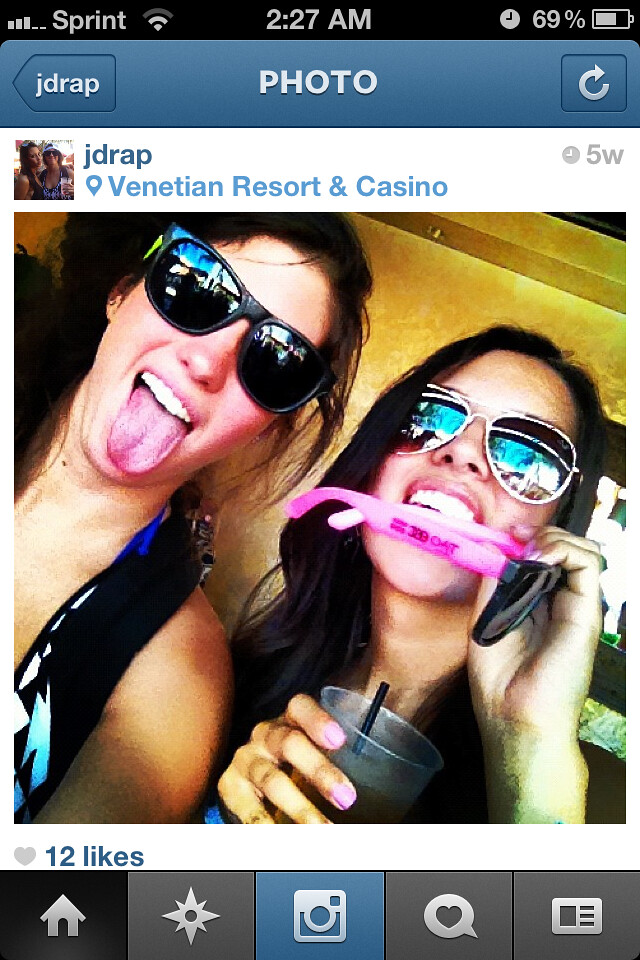This image depicts a detailed screenshot from a smartphone, captured at 2:27 a.m. with a battery level of 69%, and the phone carrier being Sprint with a 2 out of 3 bar Wi-Fi signal. At the top of the screenshot, a blue banner reads "J-DRAP Photo," with "J-DRAP, Venetian Resort and Casino, 5W" below it. The screenshot features a central photo of two Caucasian women, one with darker hair, each wearing sunglasses with blue reflections. The woman on the left is sticking her tongue out while wearing black sunglasses and a sleeveless shirt, showing a small earring. Her counterpart on the right is holding a drink with a straw and another pair of sunglasses, which she appears to be biting or holding near her mouth. The background showcases a gold, shiny wall. Below the photo, the number of likes is displayed, totaling 12 likes, followed by a navigation bar with various icons, including a house, star, camera, heart, and a text bubble.